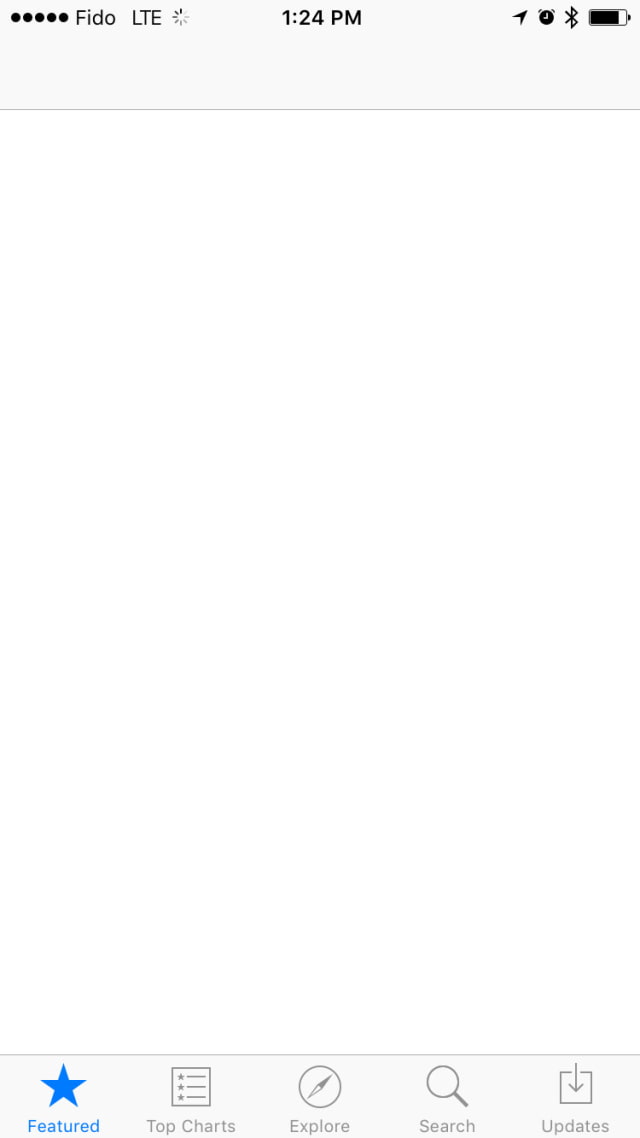The image appears to be a screenshot of a mobile device screen. At the top left corner, five dots are displayed, followed by the text "Fido" and "LTE" in capital letters. The current time is shown as 1:24 p.m. To the right, there are several icons including an alarm, location, battery percentage, and Bluetooth.

Below this status bar is a large, blank white box taking up the majority of the screen. Underneath the white box, there are five menu options with distinct icons: 

1. **Featured**: Represented by a star icon. This option is highlighted.
2. **Top Charts**: Indicated by an icon resembling a box.
3. **Explore**: Shown with a circle that looks like a compass.
4. **Search**: Depicted with the magnifying glass icon typical of search functions.
5. **Updates**: Displayed with a square and a downward-pointing arrow.

The "Featured" option is the only one currently selected, giving it a distinct highlight.